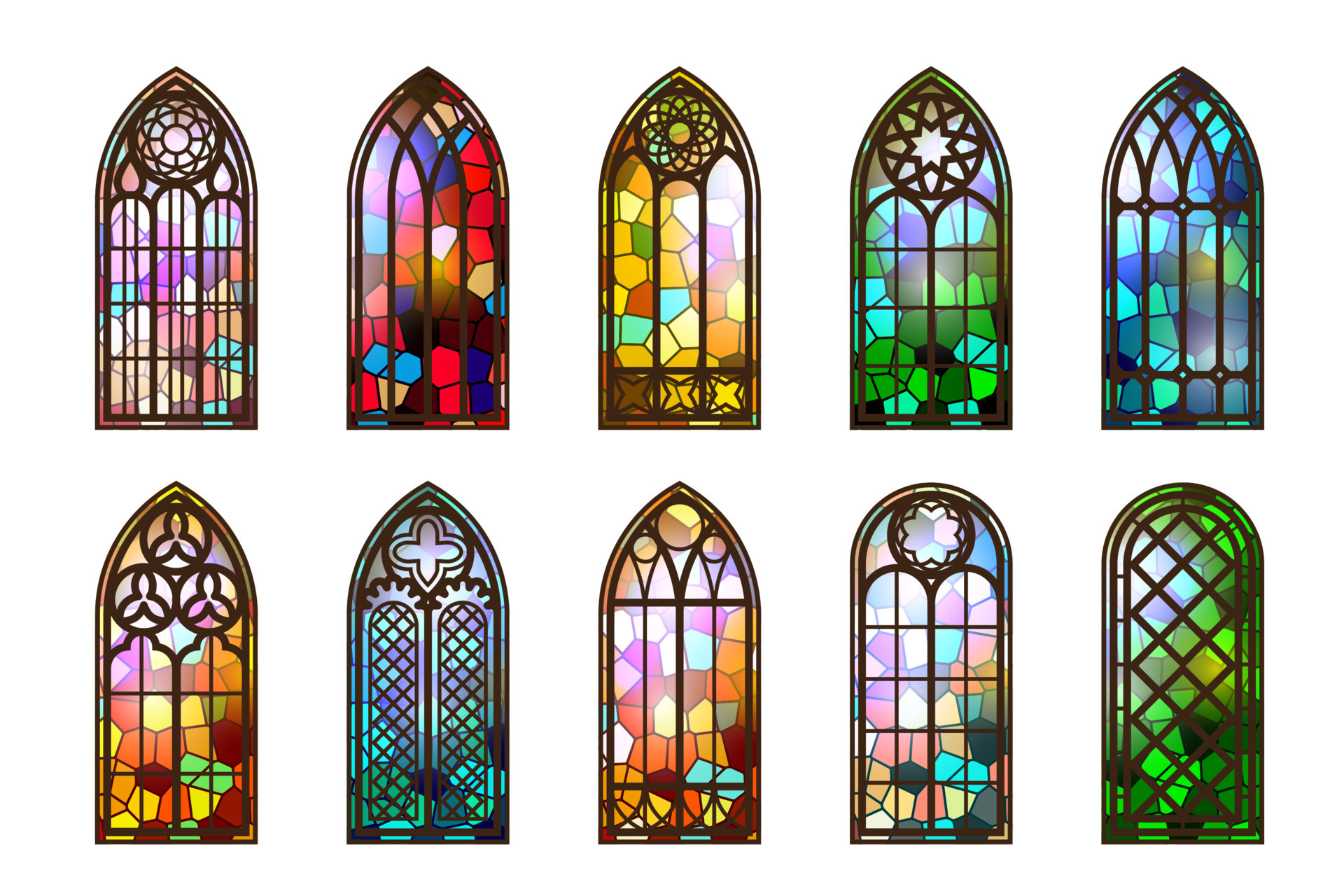The image showcases 10 distinct stained-glass windows arranged in two evenly spaced rows of five. Each window features a unique composition of colored stained-glass panels and metal grates. The windows predominantly have vertical, rectangular shapes, each topped with either a domed or arched design. The stained-glass panels exhibit a diverse palette, including greens, blues, reds, and other vibrant colors.

In the bottom right corner, a window with a circular archway is adorned with a grid-like grate, showcasing green panels behind it. The top left window features a circular design in brown, topped with three vertical sections and a rounded upper part, set against a floral stained-glass background. Adjacent to it, another window has vertical lines following its shape, filled with colors like red, white, yellow, brown, and black.

A notable window displays three interconnected circles symbolizing the Father, Son, and Holy Spirit. Another window has a lattice design, and one highlights a cross, evoking a sense of spiritual entry as if it were a gate. The intricate metal grates complement the stained-glass designs, adding layers of vertical and horizontal lines, which are typically brown, further enhancing the intricate details and rich color schemes of each window.